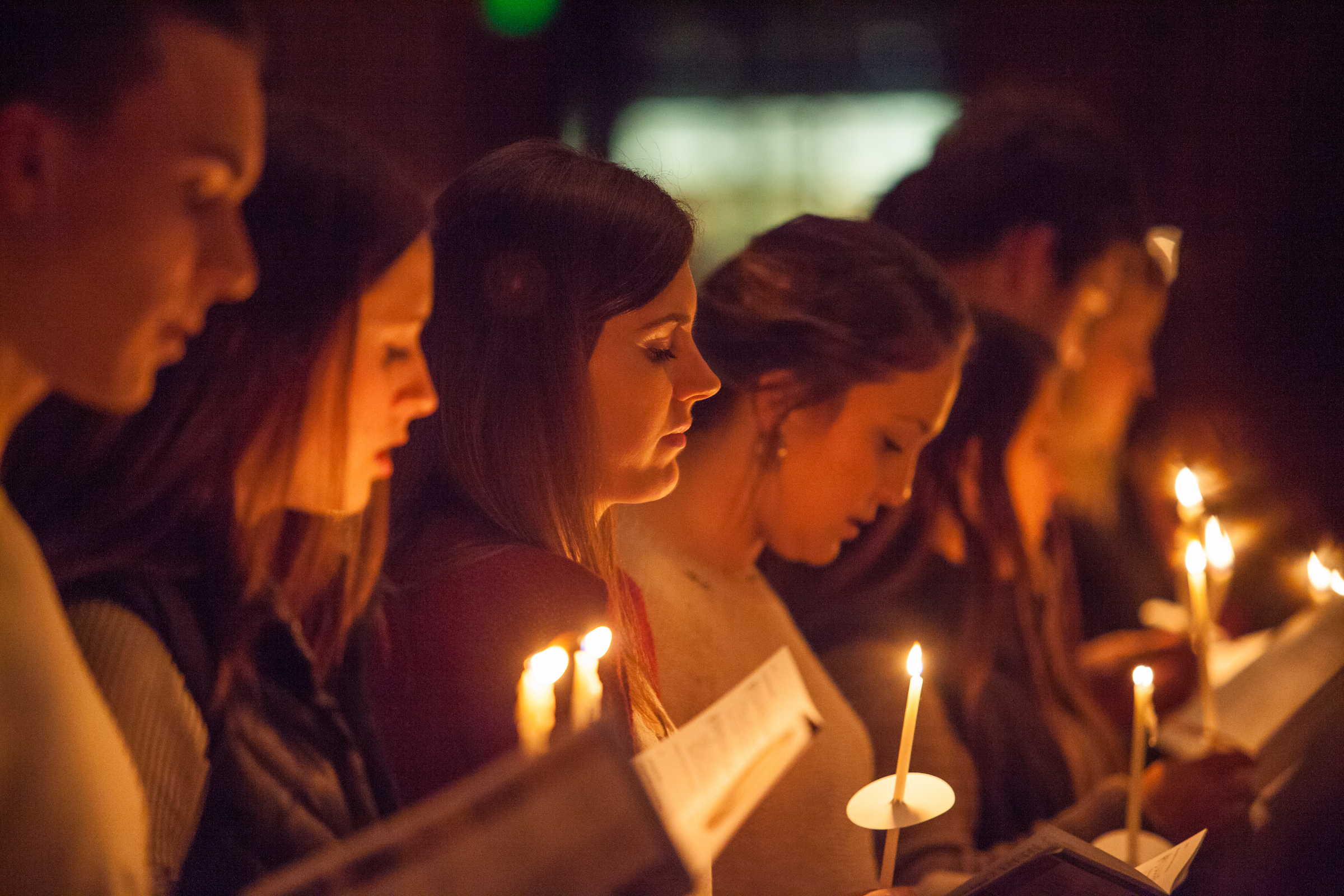In this landscape-oriented photograph, a row of men and women are seen standing closely together, participating in what appears to be a candlelight vigil. Each person holds a candle topped with a protective paper circle to catch dripping wax in one hand and a book, likely containing hymns or religious texts, in the other. The scene captures only their heads and some of their upper bodies, with all individuals looking downward at their books. The candles emit a warm white light, adding to the somber atmosphere. The background is blurred with a color theme dominated by yellowish and brown tones, suggesting a dimly lit indoor environment or nighttime setting. The overall mood conveyed is one of solemnity and reflection, as the participants engage in a shared moment of remembrance.